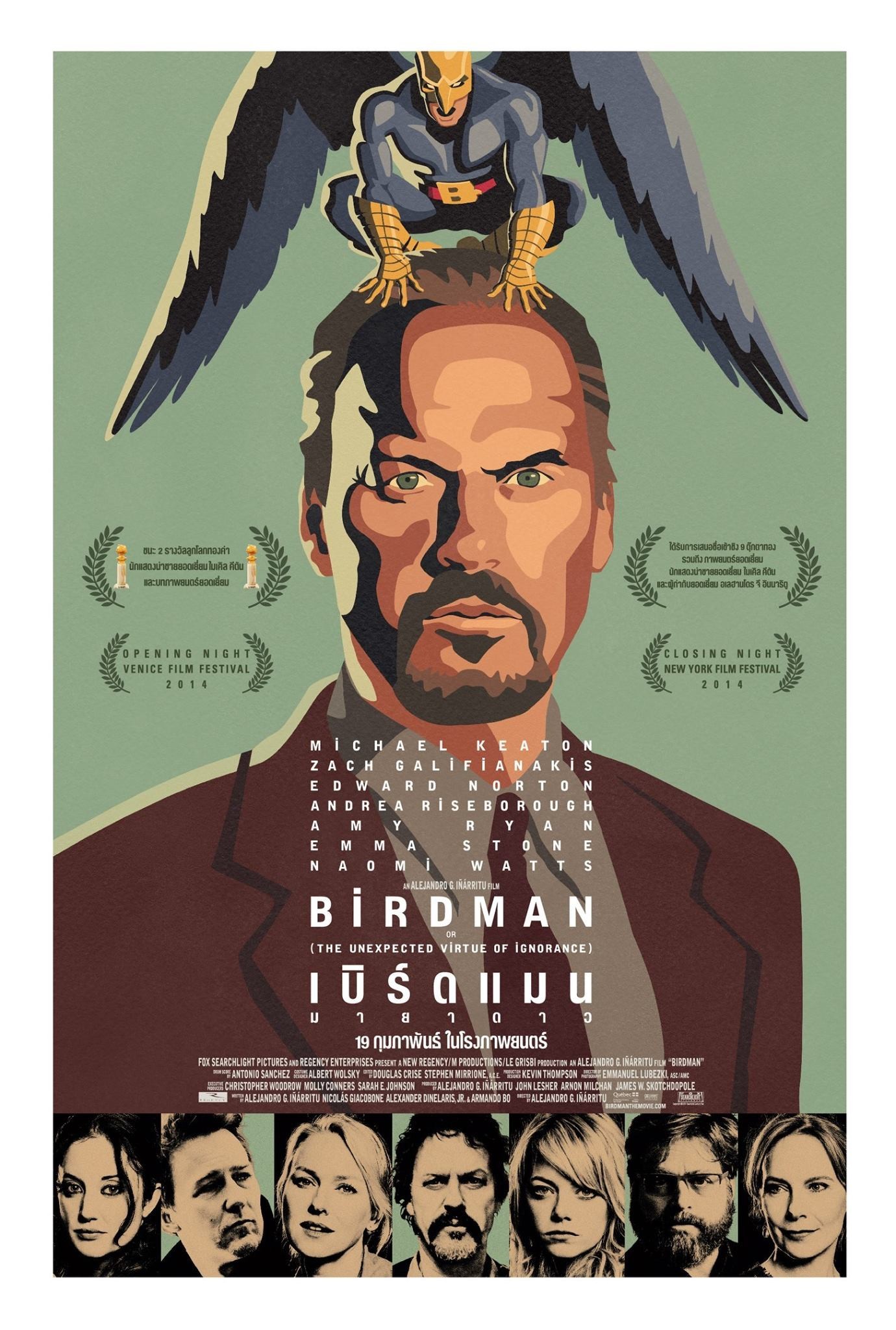This vibrant and intriguing promotional movie poster features a vividly colored pastel green background, set against which is a sharply dressed man at the center, wearing a red suit and a brown tie over a gray shirt. The man, drawn with striking detail, has alert green eyes, a rounded nose, full lips, and a brown goatee. Perched on his head is a small, superhero-like figure, clad in a blue costume with large wings, yellow gloves, a yellow mask, and a belt with a prominent "B". This blue Birdman character adds a whimsical touch to the poster. 

The largest piece of text on the image prominently displays the movie title "Birdman", with smaller text above listing the names of actors, including Michael Keaton, Edward Norton, Emma Stone, Amy Ryan, Zach Galifianakis, Andrea Riseborough, and Naomi Watts. Additionally, there are nearly invisible reviews on either side of the man's head, though too small to decipher clearly.

Towards the bottom of the image is a series of seven photographs, likely depicting the cast members mentioned. These photographs show a variety of distinct faces, adding further detail and personality to the poster. The poster also features four award-like plaques in the background, hinting at the film’s accolades. The overall style of the image, combined with the colorful ensemble and dramatic posing, makes it a compelling and eye-catching depiction for a movie titled "Birdman".